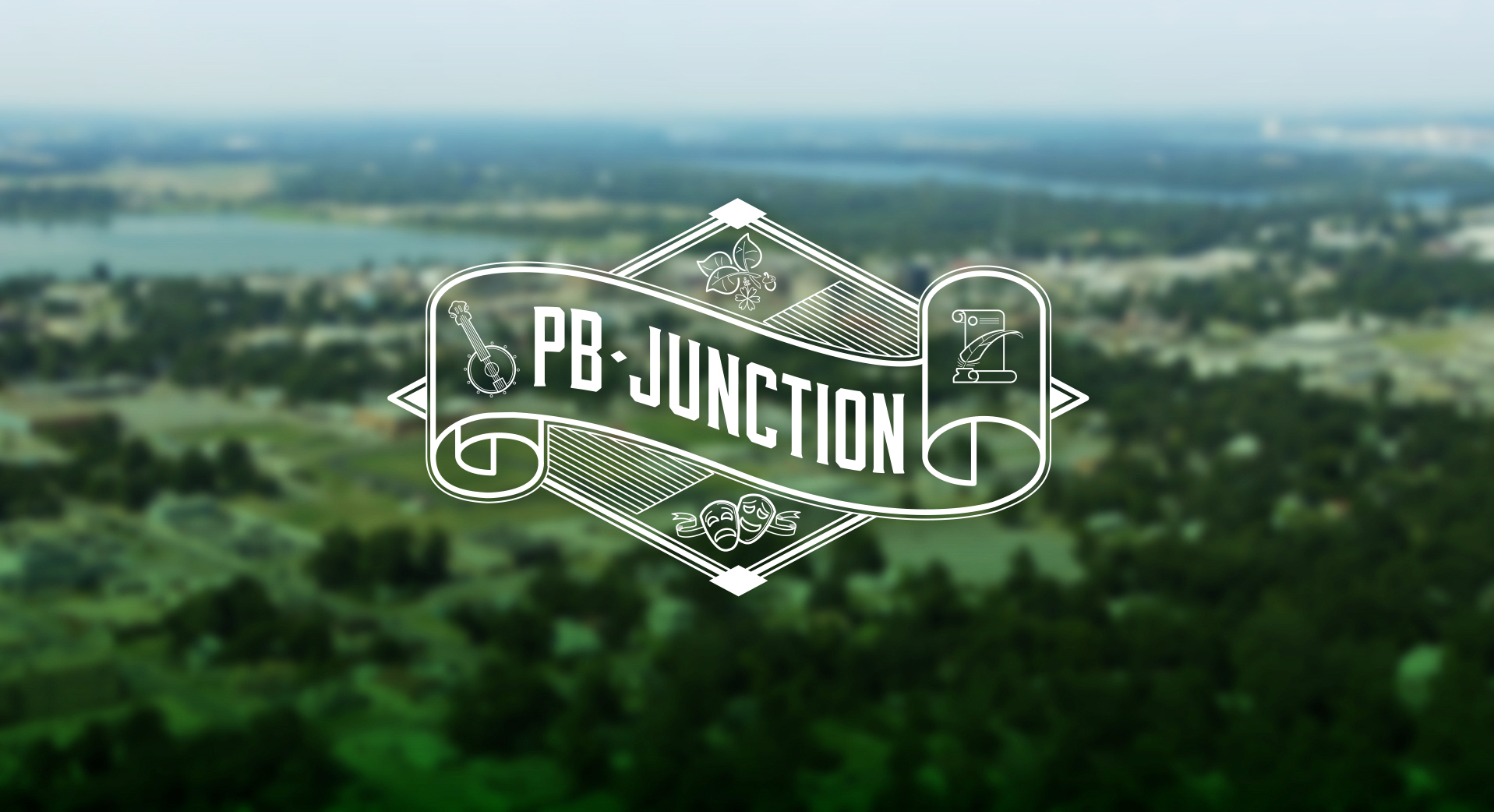The image features an aerial shot with a blurred background showcasing a green field surrounded by a dense forest. In the upper left, there's a visible body of water, presumably a lake, encased by fog and hazy clouds, creating a misty horizon. The foreground reveals a mix of dark green trees and another water body, perhaps a river. 

Dominating the center of the image is a detailed white logo for "BP Junction." The logo comprises a diamond shape in the backdrop. In front of the diamond, there's a horizontally and vertically oriented ribbon scroll—curled under on the left and over on the right. The vertical scroll on the upper right corner holds a quill pen, while the horizontal one on the left features a banjo. Beneath this intricate design are the classic happy-sad theater masks, while the top is adorned with three leaves and berries.